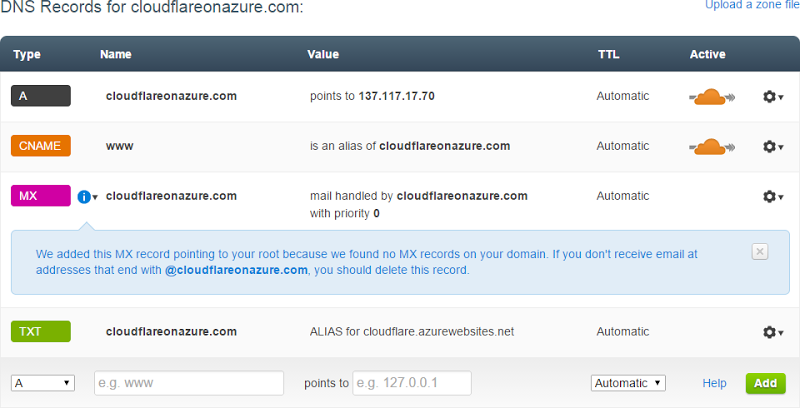The image depicts a DNS record interface for Cloudflare on azure.com. On the upper left-hand side, there is a prominent title in black font indicating "DNS Record for Cloudflare on azure.com." In the upper right-hand side, there is smaller blue text that says "Upload a zone file." Below the header section, spanning the width of the image, is a grey bar with white titles for each column. These column titles include:

1. **Type** - First column
2. **Name** - Second column
3. **Value** - Third column
4. **TTL** - Fourth column
5. **Active** - Fifth column

Directly underneath this grey bar, the first row of the DNS record is detailed. The Type is represented by the letter "A" inside a brown box. The Name column contains "Cloudflare on azure.com." The Value is listed as "2137.117.17.70," and additional columns such as TTL and Active would provide further details if visible.